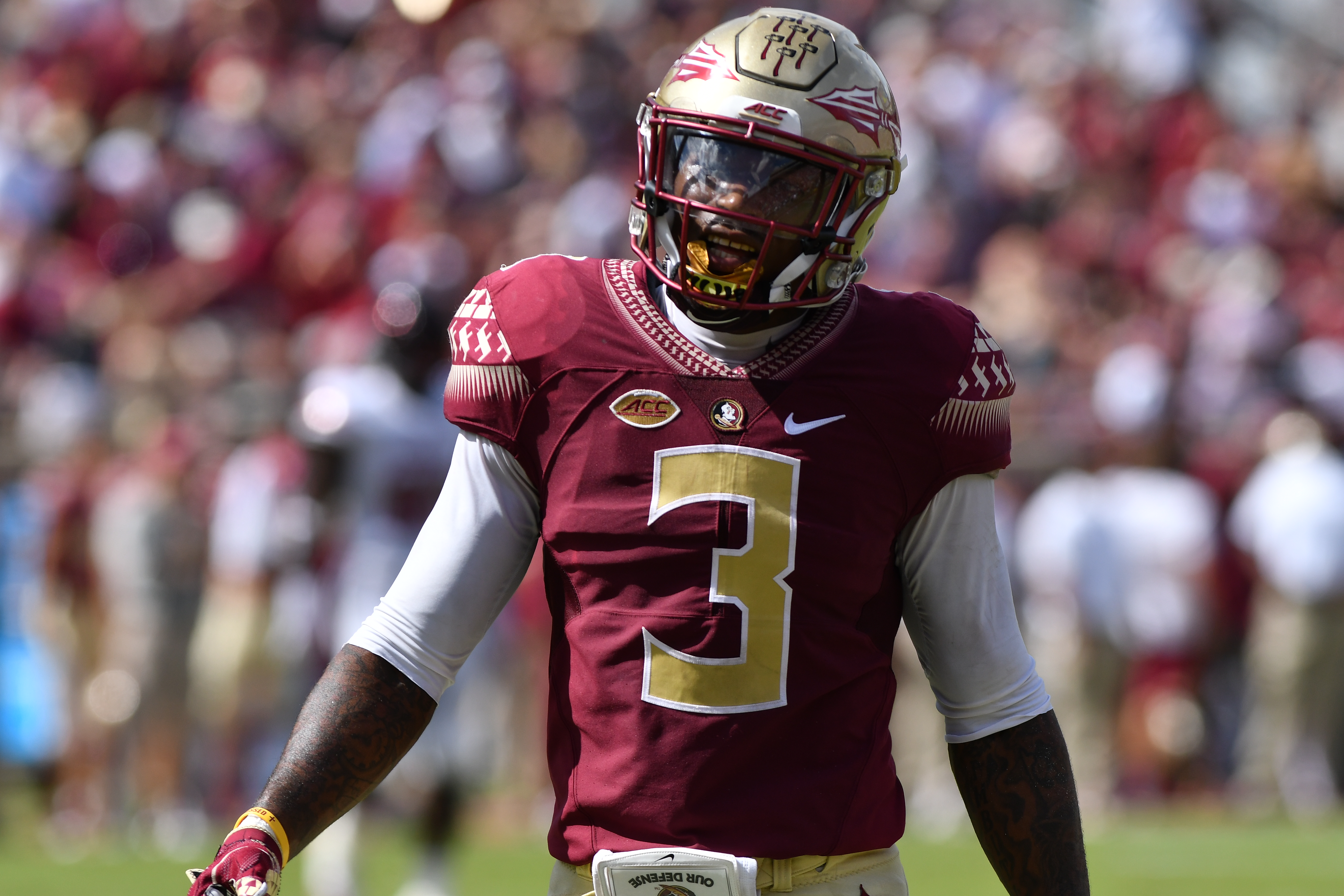This is a vibrant color close-up photograph of an African American football player, wearing the number three on his wine-colored jersey, sponsored by Nike. The foreground sharply features the player, captured from the waist up, showcasing his confident smile and gaze away from the camera. The jersey, embellished with a gold and white number three, is paired with a white, quarter-length spandex shirt underneath. His gold helmet, adorned with red, white arrows, and an ACC logo football-shaped patch, catches the sunlight, creating striking reflections and highlights. His hands are gloved in red with yellow trim. Behind him, the blurred background reveals fans and players amidst a sunny day, their attire dominated by shades of dark red, blending seamlessly into the grassy field.